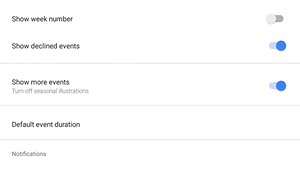Here is a clean and detailed caption for the image:

"A small square screenshot captures the settings interface of a scheduling or reminder app. At the top left, the option "Show Week Number" is visible, accompanied by a toggle switch on the right that is turned off. Below, the second option on the left reads "Show Declined Events," with its associated toggle switch turned on. A gray horizontal line separates this option from the next one, "Show More Events," which is followed by small gray text that is partly obscured, but a toggle switch to the right of it is turned on. Further down, the option "Default Event Duration" is displayed in black text without any accompanying toggle. Another narrow gray horizontal line is beneath this option, followed by the "Notifications" setting, which also lacks a toggle switch. The entire screenshot has a white background and appears to be a closely cropped section of the app’s settings menu."